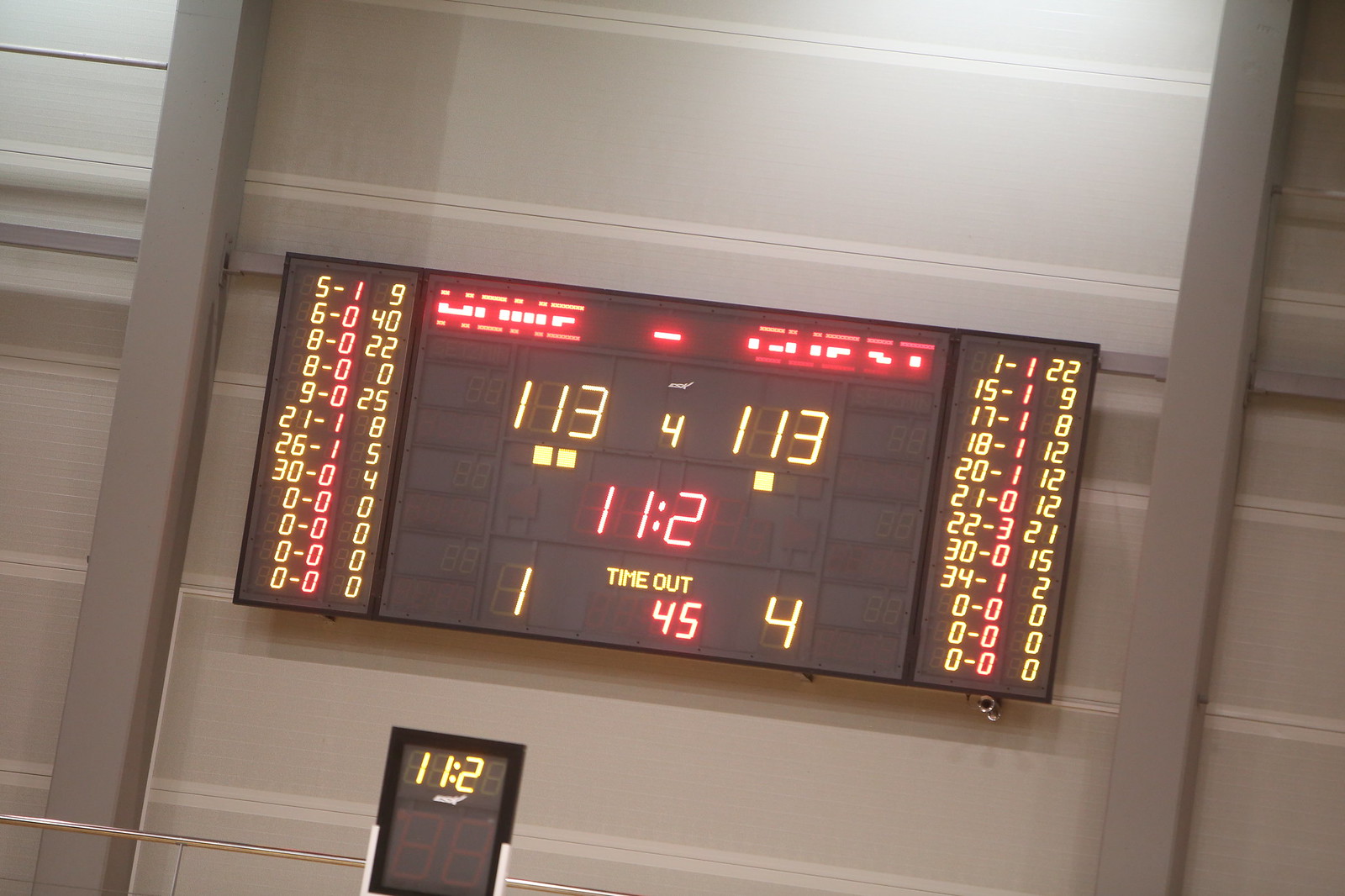The image features a black basketball scoreboard mounted on a light gray background with dark gray vertical bars, resembling a tin wall or roof. At the top center of the scoreboard, "Home" is displayed in red on the left, and "Guest" is on the right. Below these labels, the scores for both teams are shown in gold, with each team having a score of 113. In between the scores, a large red "4" signifies the fourth quarter. Under this, in pink, the shot clock reads 11.2. Below the shot clock, the timeouts are indicated: the Home team has one timeout left, while the Guest team has four. Additionally, running down the left and right sides of the scoreboard, there are lists of player numbers with their respective points scored in yellow and fouls in red.